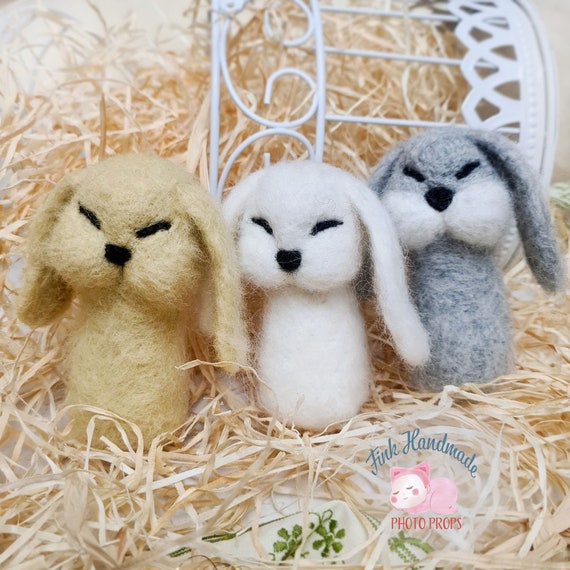Caption:  
The image features a whimsical scene centered around three felt-crafted bunnies, meticulously detailed to emphasize their fuzziness. There is a tan bunny, a white bunny, and a gray and white bunny, each with expressive black eyes and noses, giving them a lively appearance. They are nestled atop a bed of blonde-colored straw, enhancing the rustic charm of the composition. In the background, a white metallic object with intricate curly designs and lattice work adds an element of elegance. The top of the image displays a blue-font title, followed by a reddish-pink subheading. An icon of a sleeping pink creature with pointy ears and two pink spots on its face is prominently featured, adding a touch of playful whimsy. A watermark is present at the bottom of the image, ensuring credit to the creator.